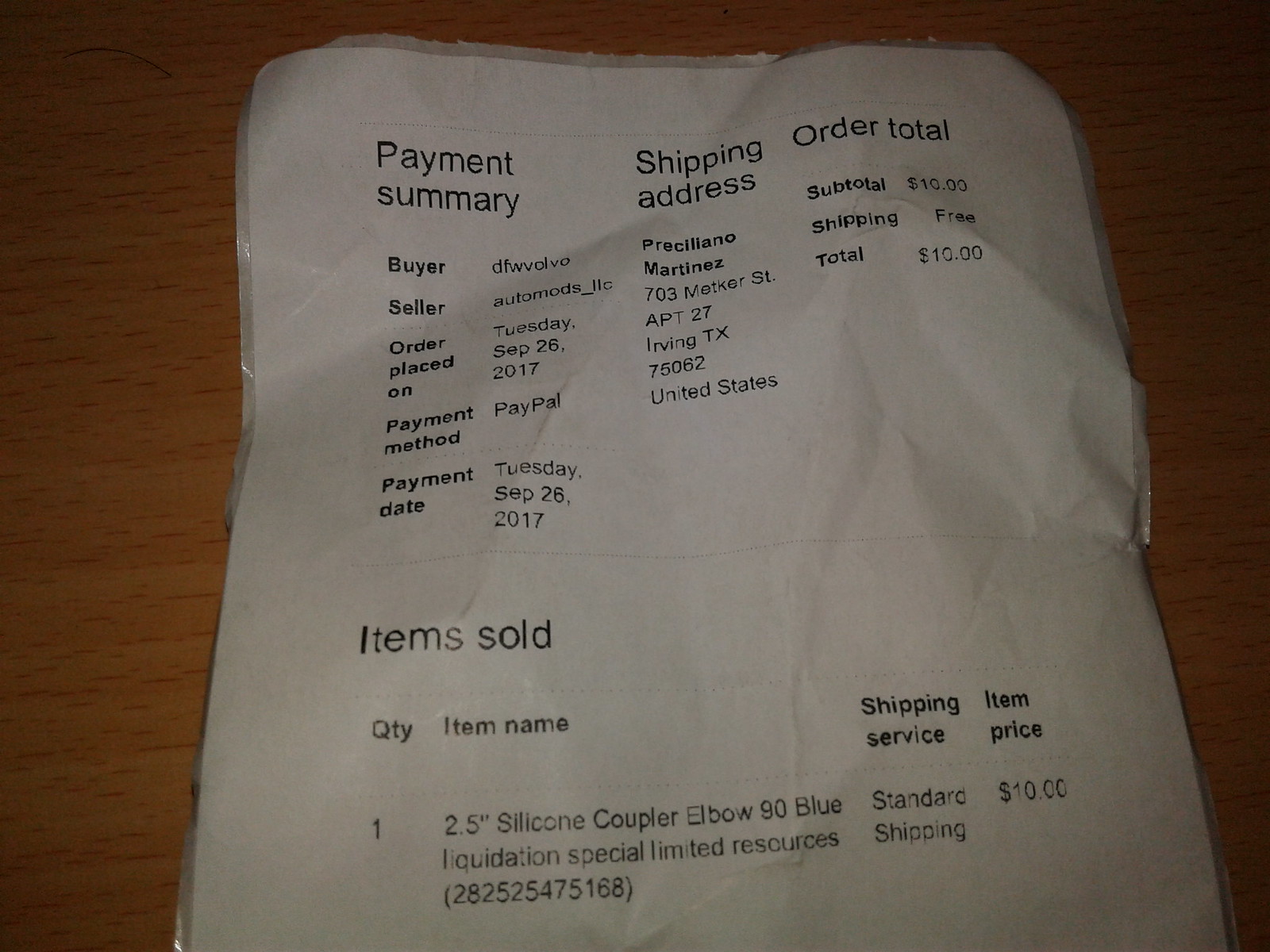This is a top-view photograph of a white receipt lying on a golden brown wooden surface. The receipt, which appears slightly crumpled, prominently features a "Payment Summary," "Shipping Address," and "Order Total" at the top. The buyer's ID is "DFWVOLVO," and the seller is "AutoMods LLC." The order was placed on Tuesday, September 26, 2017, with the payment made via PayPal on the same date. The shipping address listed is "Persolino Martinez, 703 Metcalfe Street, Apartment 27, Irving, Texas, 75062, United States." The item sold is described as a "2.5-inch Silicone Coupler Elbow, 90-degree, Blue," listed as a liquidation special under limited resources. The item price was $10, and standard shipping was free, making the total amount $10. The receipt also displays a serial number: 282525475168.